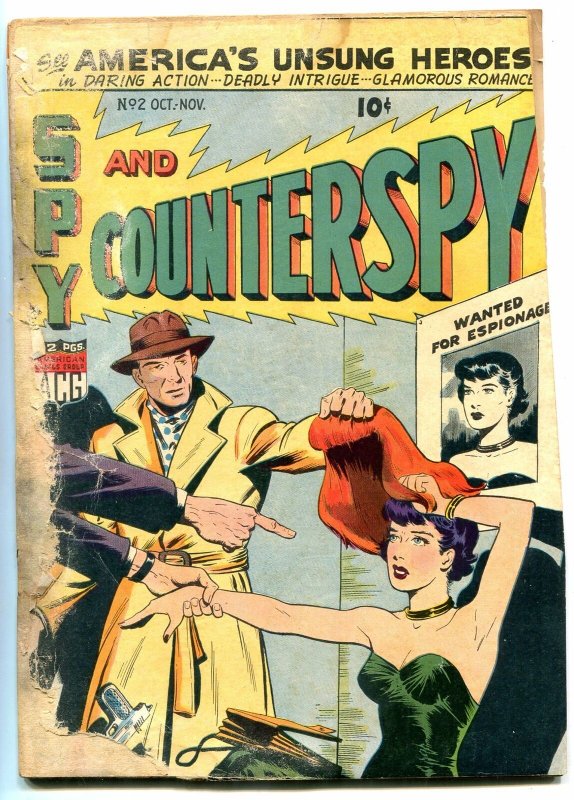This is the cover of an old, worn comic book with tattered edges. The title at the top boldly declares, "See America's Unsung Heroes in Daring Action, Deadly Intrigue, Glamorous Romance." Below that, it notes "No. 2, October - November," and the price, "10 cents," displayed alongside a zigzag arrow. The main title, "Spy, Counter Spy," is prominently printed in large green letters. The central illustration depicts a dramatic scene: a man dressed in a yellow trench coat and brown hat is pulling off a red wig from a woman seated in front of him, revealing her short blue-black hair. She is dressed in a green strapless dress and is holding onto the wig with her left hand, while her right wrist is firmly grasped by another man's hand, visible only within the frame. A gun is noticeable in the lower left corner, adding to the tension of the scene. In the background, there is a “Wanted for Espionage” poster featuring the woman's face, reinforcing her dubious character.